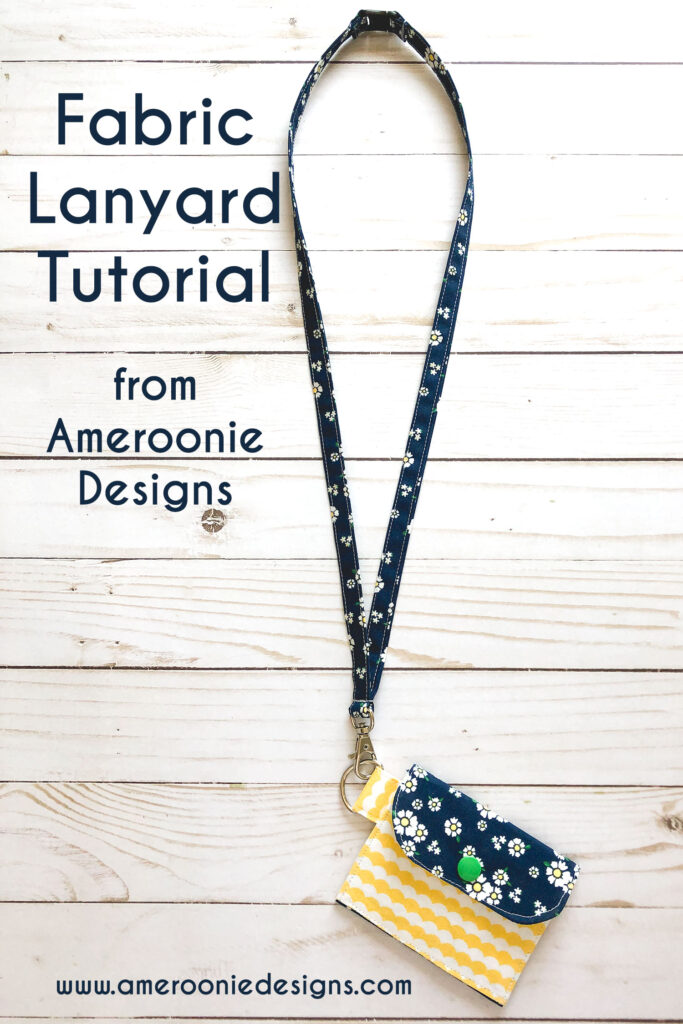The image features a detailed poster showcasing a fabric lanyard tutorial from Amaruni Designs. Hanging against a lightly-colored, horizontal wooden backdrop is a small wallet or pouch attached to a lanyard. The web address, www.amarunidesigns.com, is displayed at the bottom of the image. In dark letters to the left, the text reads "Fabric Lanyard Tutorial" with the note "from Amaruni Designs" underneath it.

The pouch itself is intricate, with a distinct design: a yellow bottom part, and a top flap that is dark blue adorned with small white flowers. It features a neon green snap button, providing a vibrant contrast. The lanyard, made of a dark blue fabric patterned with white flowers, hangs from a brass fixture attached to the pouch. The strap, approximately a foot long, starts narrow at the bottom and expands as it rises, looping through a metal ring or clasp that securely holds the pouch. The entire setup is carefully displayed on the blanched, wood-grained background, highlighting the craftsmanship and aesthetic design.